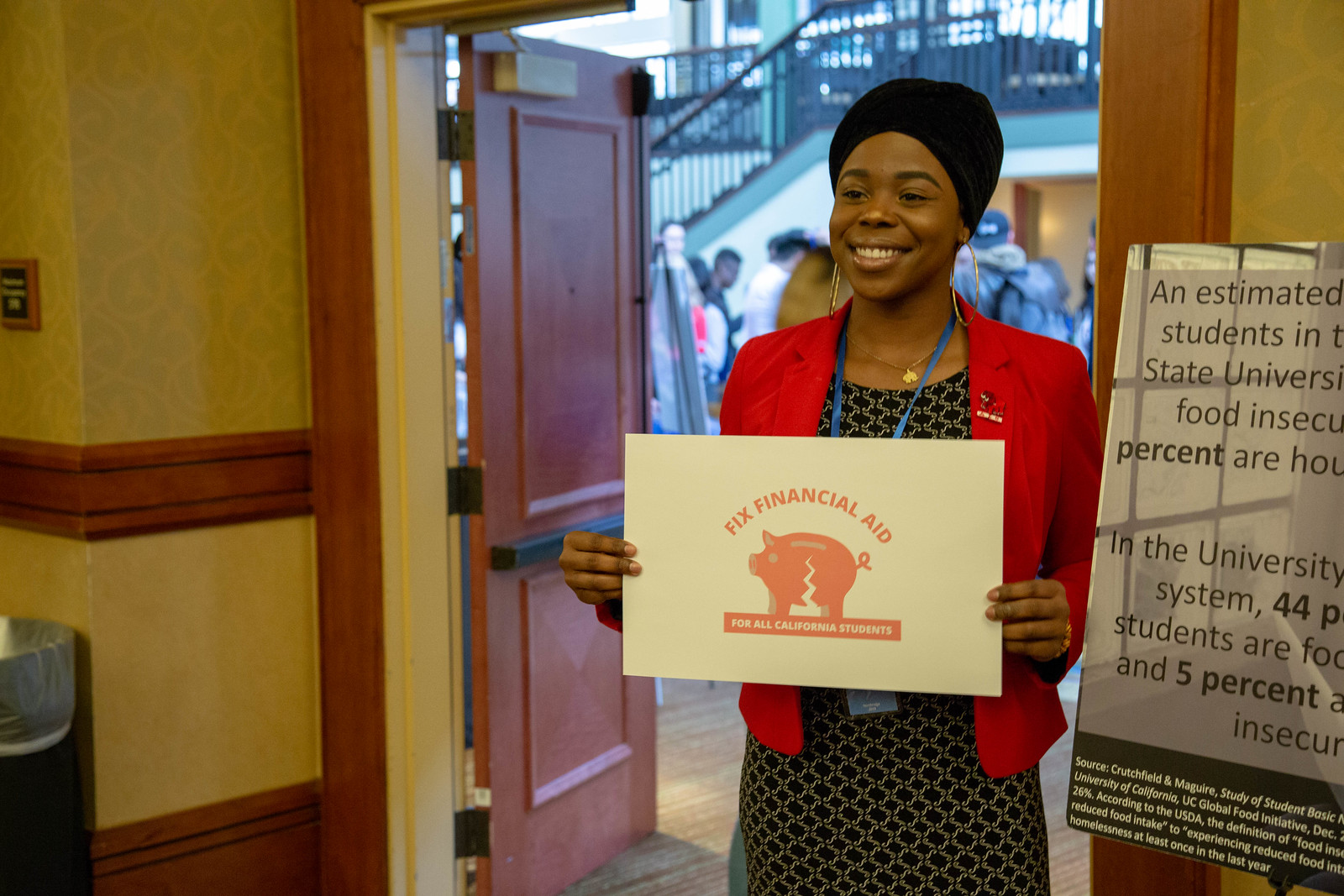This photograph features a striking young African American woman with a warm, welcoming smile. She is holding a prominent white cardboard sign with vibrant orange text that reads, "Fixed Financial Aid for All California Students," accompanied by an image of a cracked piggy bank. Dressed in a patterned black dress and a bold red blazer, she also dons a black headscarf. Around her neck, she wears a lanyard carrying a partially obscured name tag.

The setting appears to be a well-lit indoor area, possibly a school or community center. She stands just inside an open doorway, through which a bustling lobby or hallway is visible. Behind her, blurred figures navigate a staircase leading to an upper level. The walls in her room feature a two-tone design: the bottom half is beige, while the top half boasts a gold, yellowish damask wallpaper, all framed with brown wooden trim and doors.

To her left, on the image’s right side, there is a partially visible informational sign with a gray background and black text mentioning statistics about food insecurity among students in the university system, but the complete text is obscured. The environment is characterized by the contrast between the warm tones of the wood and wallpaper and the professional, yet approachable vibe of the woman's attire and demeanor.